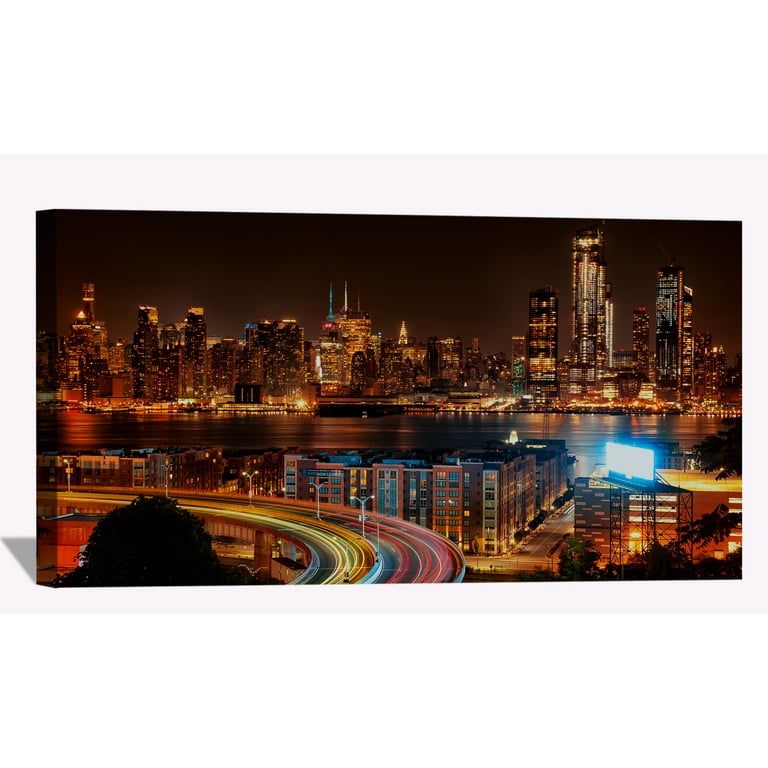The image depicts a nighttime cityscape that appears to be New York City, viewed from across a river. Centered within the slightly off-white background, the painting itself stands out roughly an inch from the wall. The top half of the artwork showcases a stunning array of commercial skyscrapers, their windows aglow with warm yellow, orange, and white lights, creating a vibrant urban skyline under a hazy night sky. Below this, a wide, dark river flows laterally across the scene, reflecting the city's lights. In the foreground, there's a more residential area with six-story apartment buildings and various smaller structures illuminated by street lamps. A notable feature is a curved highway that wraps around like branches of a tree, detailed with streaks of pink and yellow lines on the asphalt. Further, there are additional urban elements including docks, piers, and a brightly lit neon billboard, adding to the bustling city atmosphere. The detailed juxtaposition of tall skyscrapers and nearer residential buildings, all enveloped in artificial lighting, creates a dynamic and captivating nightscape.